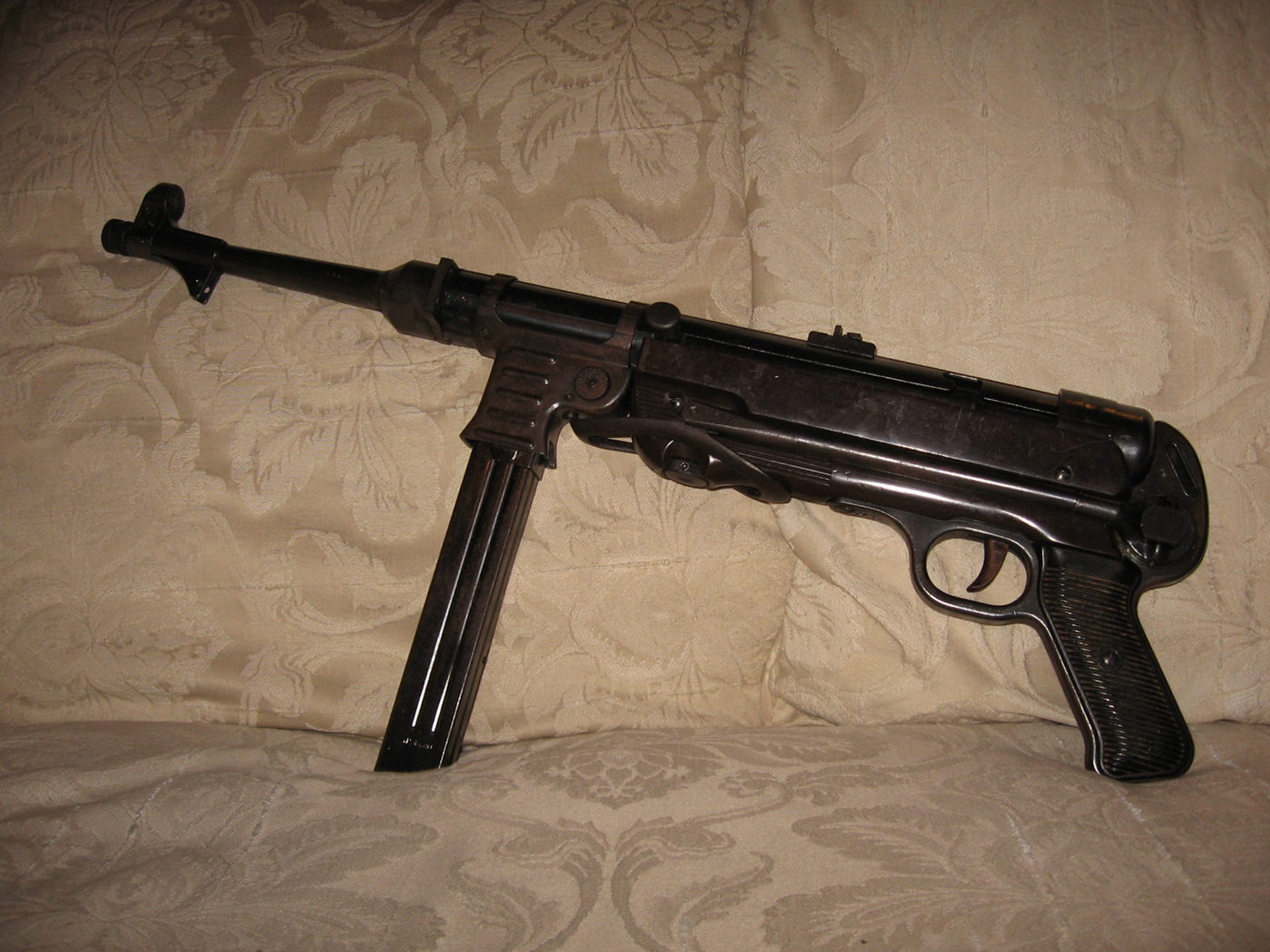This detailed photograph captures a black, possibly modified firearm positioned prominently in the center of the image. The gun, which resembles an old-time rifle with a long barrel and additional section, features a standard pistol-type handle and an extra front grip, possibly accompanied by an extended attachment like a silencer. It's mounted on a stand for display. The background consists of a plush surface, either a couch or bed, adorned with shiny beige or light brown cushions featuring intricate paisley and floral designs. The contrast between the elegant fabric texture and the austere black metal of the gun creates a striking visual.